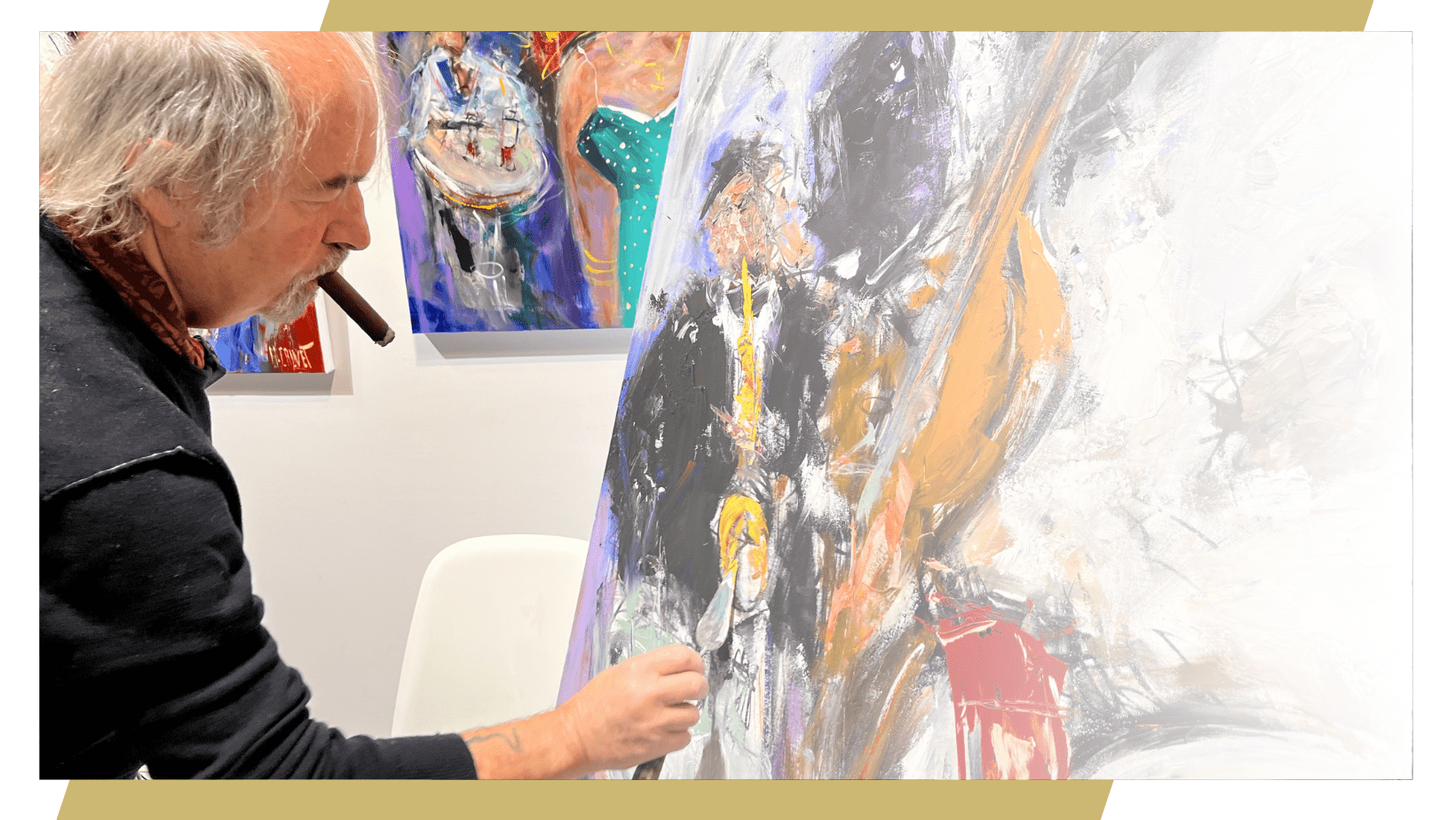An older gentleman, bald on the top with long gray hair on the sides, is deeply absorbed in his art. Clad in a black sweater over a red collared undershirt, he has a lit cigar hanging from the left side of his mouth. He's meticulously applying paint with a putty knife to a canvas featuring an abstract scene. The painting depicts a black-suited man wearing a black hat and playing a yellow saxophone, his silhouette casting a shadow that blends into another angular humanoid figure playing a large instrument resembling a cello. The dynamic background of the painting is a subtle interplay of bold reds, whites, blacks, and purples.

Behind the artist hang two more abstract paintings. The one to the right depicts a fantastical scene involving a Martian-like astronaut in a white suit and a green-faced humanoid stormtrooper. The artwork on the left, partially obscured by the artist, hints at vibrant blue and red tones. Additionally, under the man's distinctive facial features and the tip of his beard, another barely visible painting features a woman in an aqua dress standing next to a drummer, evoking a musical theme echoed in the primary work.